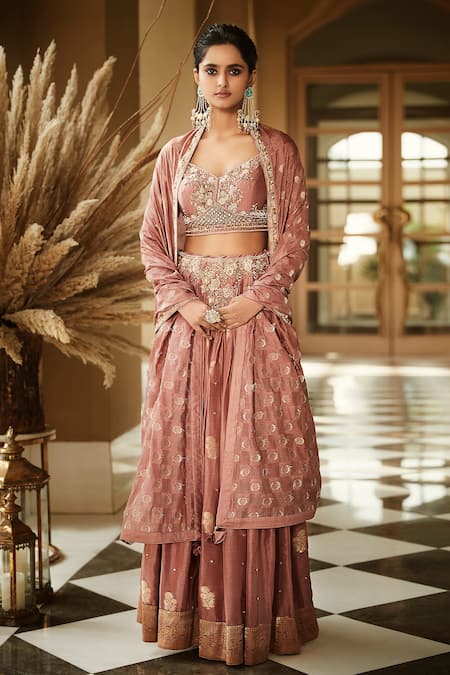The image features a young Indian woman standing elegantly in a hall with a distinctive black and white checkerboard floor that leads towards a brass double door with window panels. The hall has brown walls adorned with decorative elements, including a pillar and a vase containing dried wheat sheaves. The woman, with her dark hair either put up or cut short, has a serene expression as she gazes directly at the camera. She is adorned with large, elaborate earrings featuring silver tangents and multiple pieces of jewelry.

Her attire is a detailed ensemble consisting of a revealing bralette and a long, salmon-pink layered skirt that reaches her ankles. The bralette, embellished with light gold and white embroidery, exposes her midriff. She wears a matching shawl that drapes over one arm and extends to the length of her skirt. The ensemble is further embellished with intricate white, pearly, and silvery decorations along the edges and fringes. Her hands, positioned in front of her, display a prominent ring. The overall look is both traditional and contemporary, with meticulously embroidered floral patterns and gold accents adding a touch of opulence to her attire.